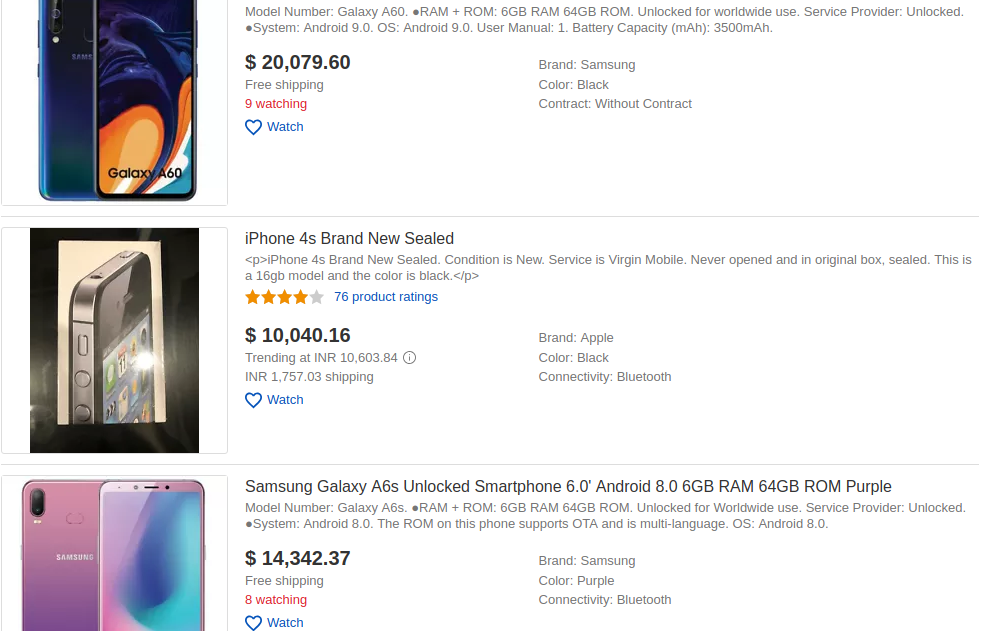Here is the cleaned-up and detailed caption for the screen capture of the shopping website:

---

**Screen Capture from a Shopping Website Featuring Smartphones**

1. **Samsung Galaxy A60**:
   - **Image**: Shows the back of a metallic blue Samsung Galaxy A60 with a vibrant, multi-colored wallpaper in navy, orange, teal, and white.
   - **Details**:
     - **Model Number**: Galaxy A60
     - **RAM/ROM**: 6GB RAM / 64GB ROM
     - **Compatibility**: Not for worldwide use, service provider unlocked
     - **Operating System**: Android 9.0
     - **Battery Capacity**: 3500mAh
     - **Price**: $20,079.60
     - **Shipping**: Free
     - **Watchers**: 9 people watching
     - **Brand**: Samsung
     - **Color**: Blue
     - **Contract**: Without contract
   
2. **Apple iPhone 4S**:
   - **Image**: Displays an unopened iPhone 4S box containing a bulky silver and black cell phone.
   - **Details**:
     - **Condition**: Brand new, sealed, never opened
     - **Service Provider**: Virgin Mobile
     - **Storage**: 16GB
     - **Price**: $10,040.16 (Trending at INR 10,603.84)
     - **Shipping**: INR 1,757.03
     - **Ratings**: 4 stars from 76 product ratings
     - **Watchers**: Button for watchers
     - **Brand**: Apple
     - **Color**: Black
     - **Connectivity**: Bluetooth

3. **Samsung Galaxy A6S**:
   - **Image**: Showcases a lavender Samsung Galaxy A6S with views of the back and a colorful wallpaper featuring pink, purple, blue, and teal.
   - **Details**:
     - **Model Number**: Galaxy A6S
     - **RAM/ROM**: 6GB RAM / 64GB ROM
     - **Compatibility**: Unlocked for worldwide use
     - **Operating System**: Android 8.0
     - **Special Features**: ROM supports OTA and is multi-language
     - **Price**: $14,342.37
     - **Shipping**: Free
     - **Watchers**: 8 people watching
     - **Brand**: Samsung
     - **Color**: Purple
     - **Connectivity**: Bluetooth